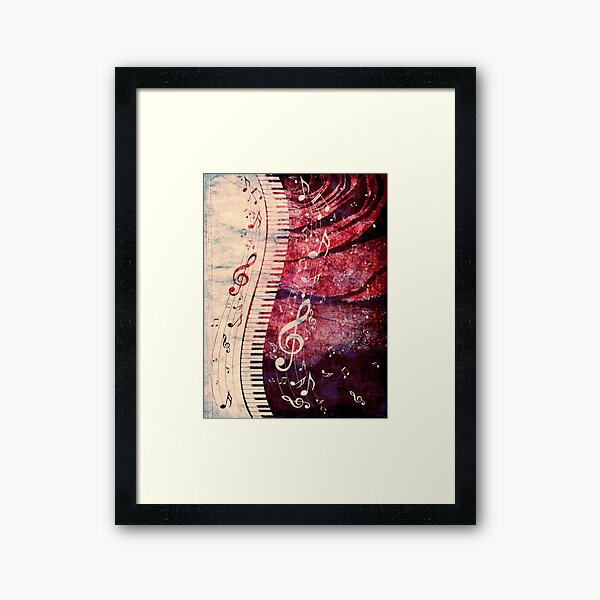This is a photograph of a framed artwork featuring a dynamic musical theme. The solid black matte frame encases a large off-white matting, creating a bold contrast with the vibrant colors of the print inside. The central image spans approximately 8 by 10 inches and showcases a rich gradient from beige on the left to deep maroon and red on the right. A curving, almost serpentine piano keyboard winds vertically through the center, composed of white and darker keys intertwined with the vibrant colors. On the left side, musical notes in red appear against the lighter background, while the right side of the image hosts beige notes amidst a backdrop of dark reds and maroons. The right portion also hints at a textured element, resembling rose petals in maroon and black, adding depth and intrigue to the overall composition. The combination of intricate musical symbols and the striking color gradient creates a captivating visual harmony.